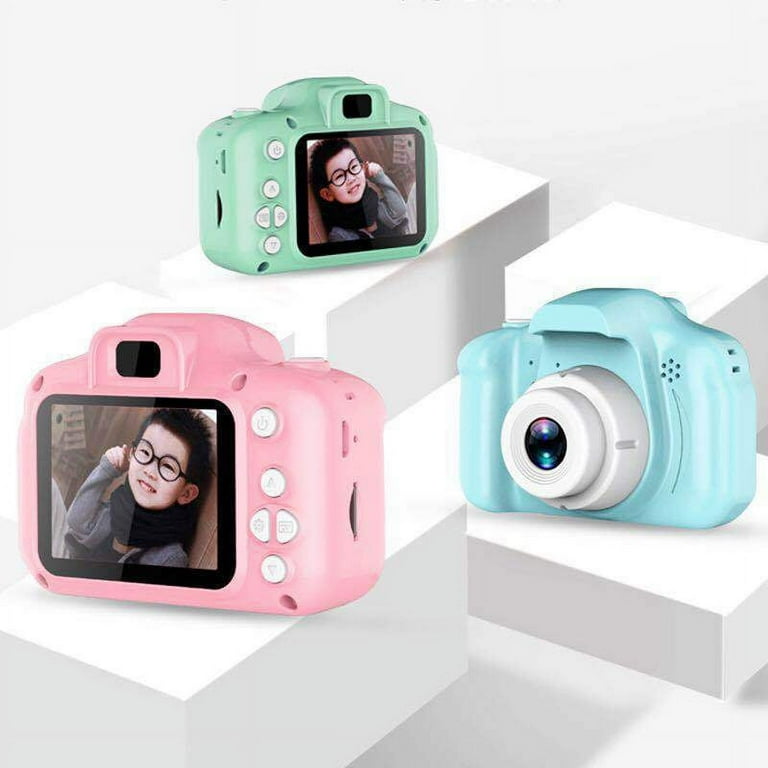This image showcases three small, colorful digital cameras designed specifically for children, likely for advertisement purposes. The cameras are perched upon layered white pedestals, creating a tiered display. Each camera comes in a distinct pastel color: teal aqua green, coral-ish light pink, and mint blue. 

The green camera is positioned at the uppermost pedestal, revealing its backside. It features an array of five white operational buttons located on the left-hand side, along with a viewing area and an actual screen that displays a photograph of a young Asian boy wearing round glasses. Below the green camera sits the pink one, similarly showing its backside. Its five functional buttons, also white, are situated on the right side. The screen similarly displays an image of the same young boy, suggesting it is the same photo. 

Finally, the mint blue camera is situated on the rightmost pedestal, facing the viewer. This allows us to see its front facade and white zoom lens prominently. All three cameras, with their distinct yet complementary pastel color schemes and simple button layouts, are clearly designed to be appealing and manageable for children.